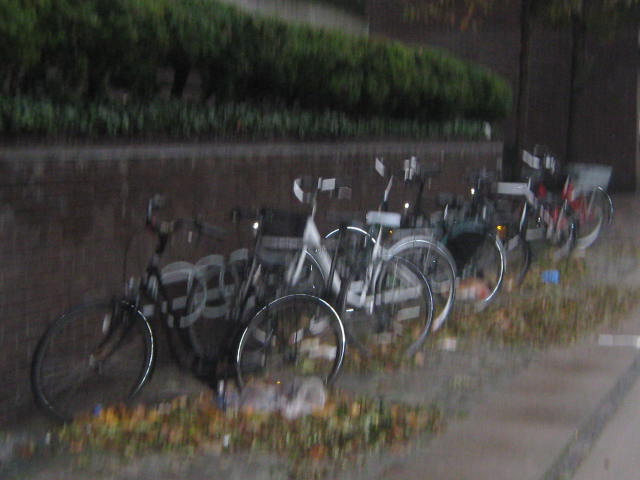This blurry photograph, taken during the day, depicts six bicycles parked in a bike rack against a tall brick wall. The wall, predominantly brown with a small line of gray brick, is topped with a dense row of dark green hedges. In front of the wall, the bicycles, which include black, white, silver, and red models, are aligned parallel to the bike rack. The bike rack itself has white loops for securing the bicycles. The ground is primarily a gravel path interspersed with patches of grass and weeds, some of which contain scattered plastic and trash. There are multicolored leaves—yellow, brown, and orange—strewn among the patches of grass. In the top right corner, the overhanging leaves of a tree are visible. Additionally, a blurry silver object, likely a trash can, is noted toward the back corner.